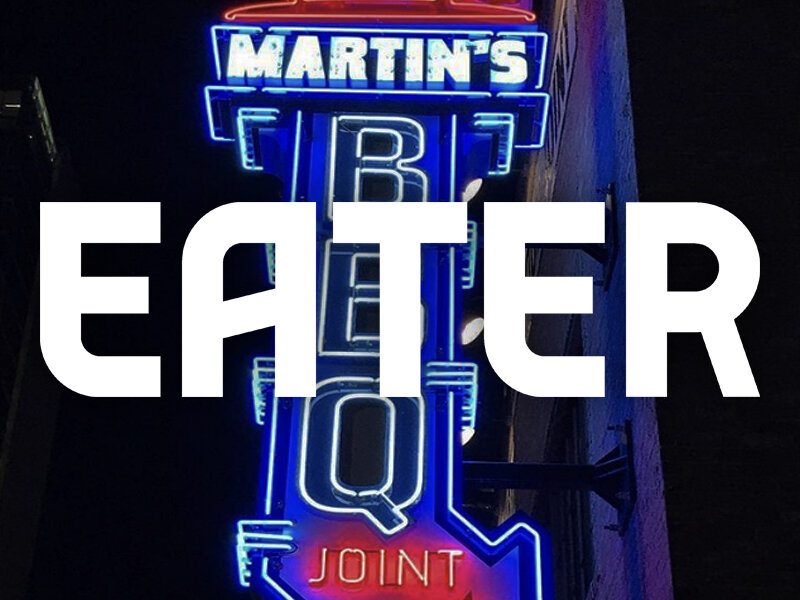This detailed photograph, likely taken at night, showcases a neon sign for Martin's Barbecue Joint, mounted on the side of a brick building. The prominent sign features "Martin's" in large blue neon letters, vertically oriented "BBQ," and "Joint" illuminated in red neon at the bottom. A portion of red neon lights at the top is cropped off. The entire scene is framed against a black sky, emphasizing the glowing neon hues. Overlaying the photo are large, bold white letters that spell "EATER." The sign is bolted to the wall in two places, and the angle of the shot suggests it was captured from a sidewalk perspective, possibly for advertising purposes. The vibrant colors and nighttime setting make the sign's illumination stand out vividly against the dark backdrop.